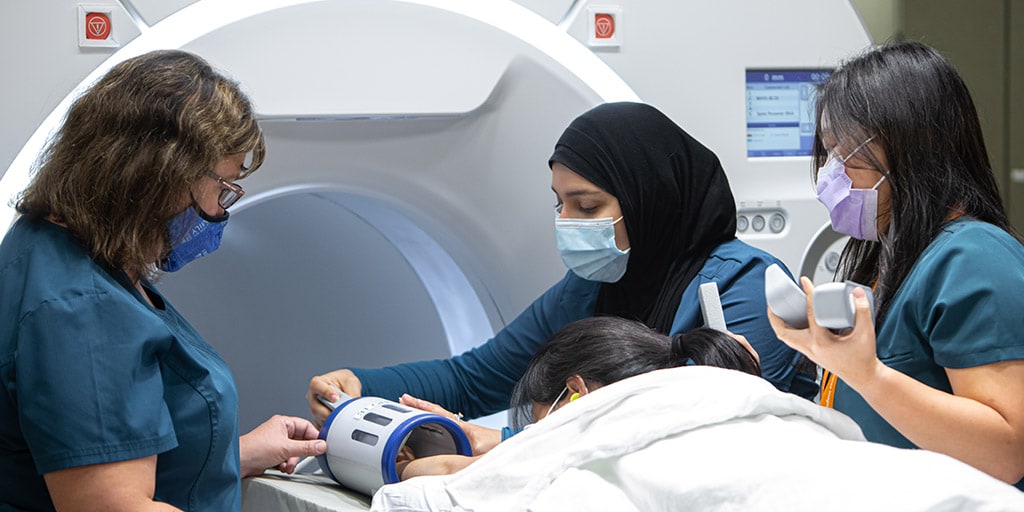Inside a medical facility, we see three female healthcare professionals, all clad in teal scrubs and personal protective equipment face masks, attending to a patient. One of the professionals wears a black hijab, another has glasses, and the third appears to be of Asian descent. The scene is set around a large, cylindrical MRI machine, predominantly white with a screen attached to its right side displaying some kind of information. Positioned face down on the gurney, the patient has black hair tied in a ponytail and is partially covered with a white blanket. Her left hand is being placed into a circular tube-like device bordered in blue, suggesting she’s undergoing a scan or test. The team appears focused on properly positioning her for the upcoming MRI scan.